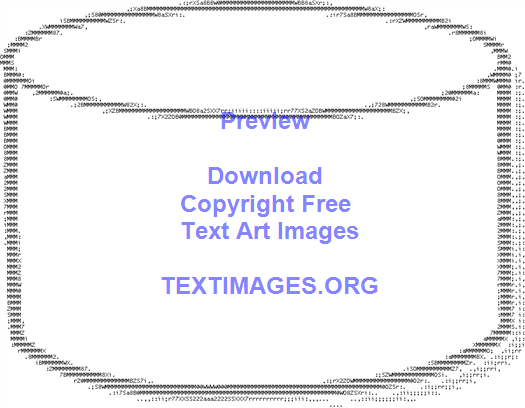The image features a predominantly white background devoid of any headers, footers, or borders, creating a minimalist appearance. Central to the image is a striking 3D cylindrical shape crafted from a myriad of black random code characters, numbers, and letters. The cylinder, which is wider than it is tall and viewed from an angle, gives a sense of depth with a long oval depicting its top surface. Superimposed on the cylinder, the word "PREVIEW" appears prominently in a red and purple hue at the top part of the shape. Below it, in the center of the cylinder, the text "Download Copyright Free Text or Images" and "textimages.org" is displayed in all capitalized purple font. The intricate design merges both artistic creativity and informative text, presenting a unique blend of digital art and text-based content. The overall aesthetic is one of clean simplicity, highlighted by the contrast between the black characters of the cylinder and the colorful inscriptions.